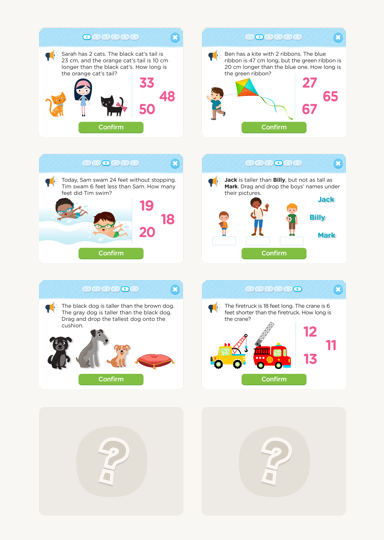The image is organized into two columns, each containing two rows. Here's a detailed breakdown of each section:

1. The top-left section features a card that reads: 
   "Sarah has two cats. The black cat's tail is 23 centimeters long, and the orange cat's tail is 10 centimeters longer than the black cat's. How long is the orange cat's tail?" 
   On the right side of the card, there are three possible answers displayed in pink: 33, 48, or 50. Below the answers is a green "Confirm" button. The image also shows a girl and her two cats.

2. The top-right section displays a card with the message:
   "Ben has a kite with two ribbons. The blue ribbon is 47 centimeters long, but the green ribbon is 20 centimeters longer than the blue one. How long is the green ribbon?" 
   To the right, the possible answers 27, 65, and 67 are listed in blue. A blue "Confirm" button is placed below the answers. The accompanying image shows a little boy flying a kite.

3. The bottom section on the left side includes another card stating: 
   "Today, Sam swam 24 feet without stopping. Tim swam 6 feet less than Sam. How many feet did Tim swim?" 
   Displayed to the right are the potential answers in pink: 19, 18, and 20, alongside a green "Confirm" button. An illustration of two boys swimming in water accompanies this card.